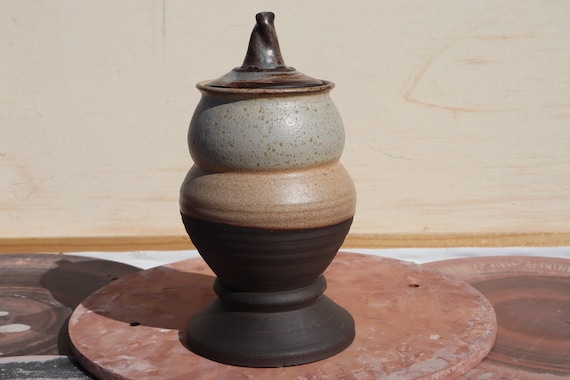The image is a detailed, up-close shot of a lidded jar pottery piece, prominently positioned in the center. The jar has a distinctly curved, multi-bulbous shape, starting with a wide, fluted base that narrows, then widens into a pronounced larger bulb before tapering slightly and culminating in a lid with a pointed top reminiscent of a witch's hat. The lid is a darker brown, while the sections of the jar transition through a palette of stone gray with tan flecks, tan, and dark brown as you move towards the base. Surrounding the jar is a circular terracotta plate, accompanied by two other platters on either side. The backdrop features a rustic whitewashed wood wall that extends upwards, showcasing its grain and subtle brown swirls. The entire scene is further accentuated by the pottery piece sitting on what appears to be a heavy tan clay or terracotta slab, highlighting its central importance in the composition.